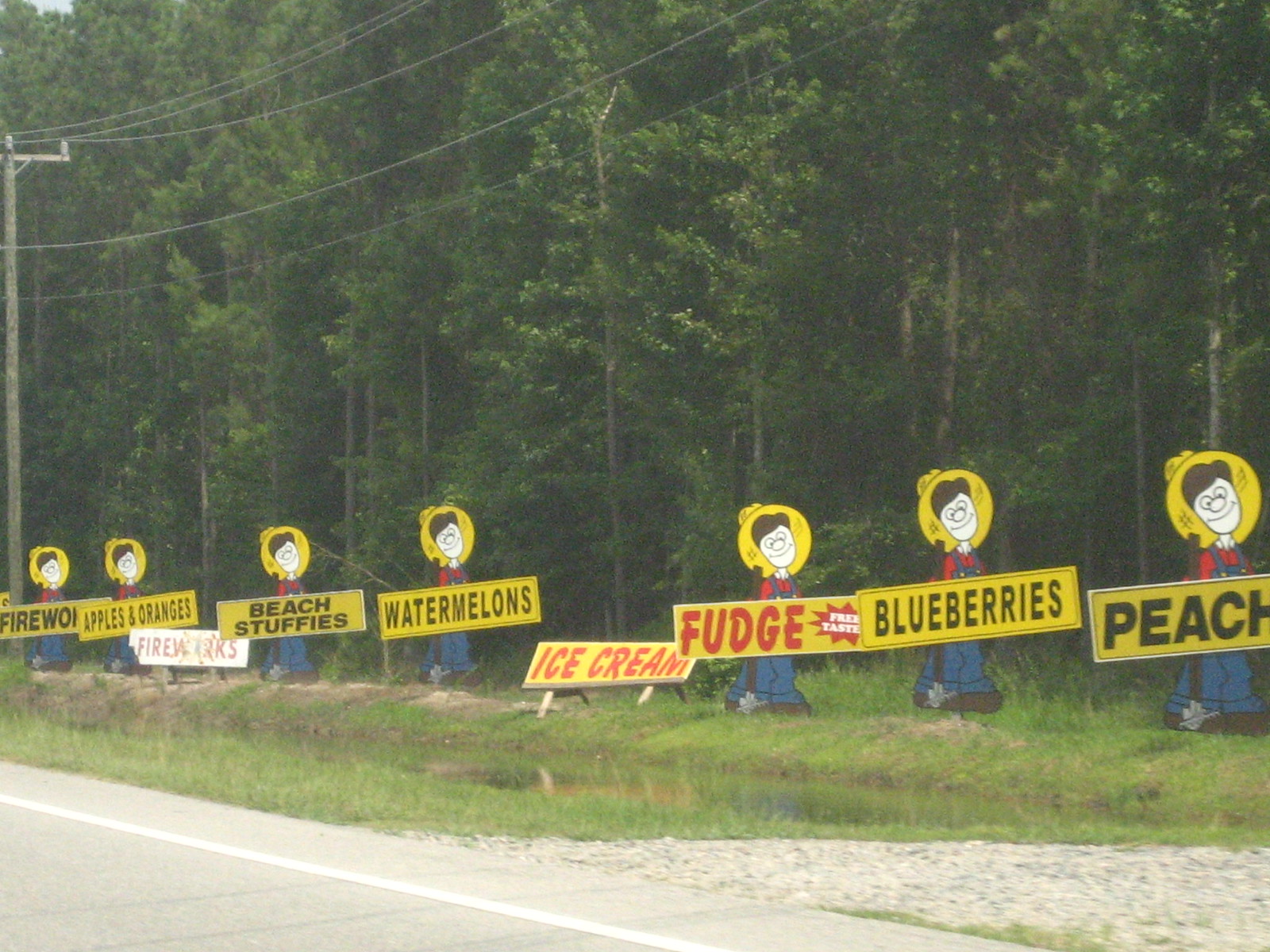In the image, there is a rural roadside scene featuring an assortment of signs. The setting includes a main road bordered by a gravel strip, which could serve as either a parking area or a secondary road. Adjacent to the gravel strip is a small pond, framed on the right by a grassy expanse leading into a dense forest. 

Standing prominently by the roadside are several whimsical cutout figures, each depicting a character wearing a yellow hat, a red shirt, and blue overalls. Their faces are sketched with a tilted expression, adding a playful touch to the display. Each figure holds up a sign with varying messages. The first cutout advertises "Peach" and "Blueberry," while the second mentions "Blueberries." Another sign promotes "Fudge - Free Taste," and yet another reads "Ice Cream," which is placed on a standalone post rather than held by a cutout figure.

Further behind, additional cutout figures display signs for "Watermelons," "Peach Stuffies," and "Apples and Oranges." In the far background, one final sign boldly advertises "Fireworks." The overall scene is vibrant and inviting, effectively capturing the essence of a countryside market or roadside stand with a diverse array of goods.